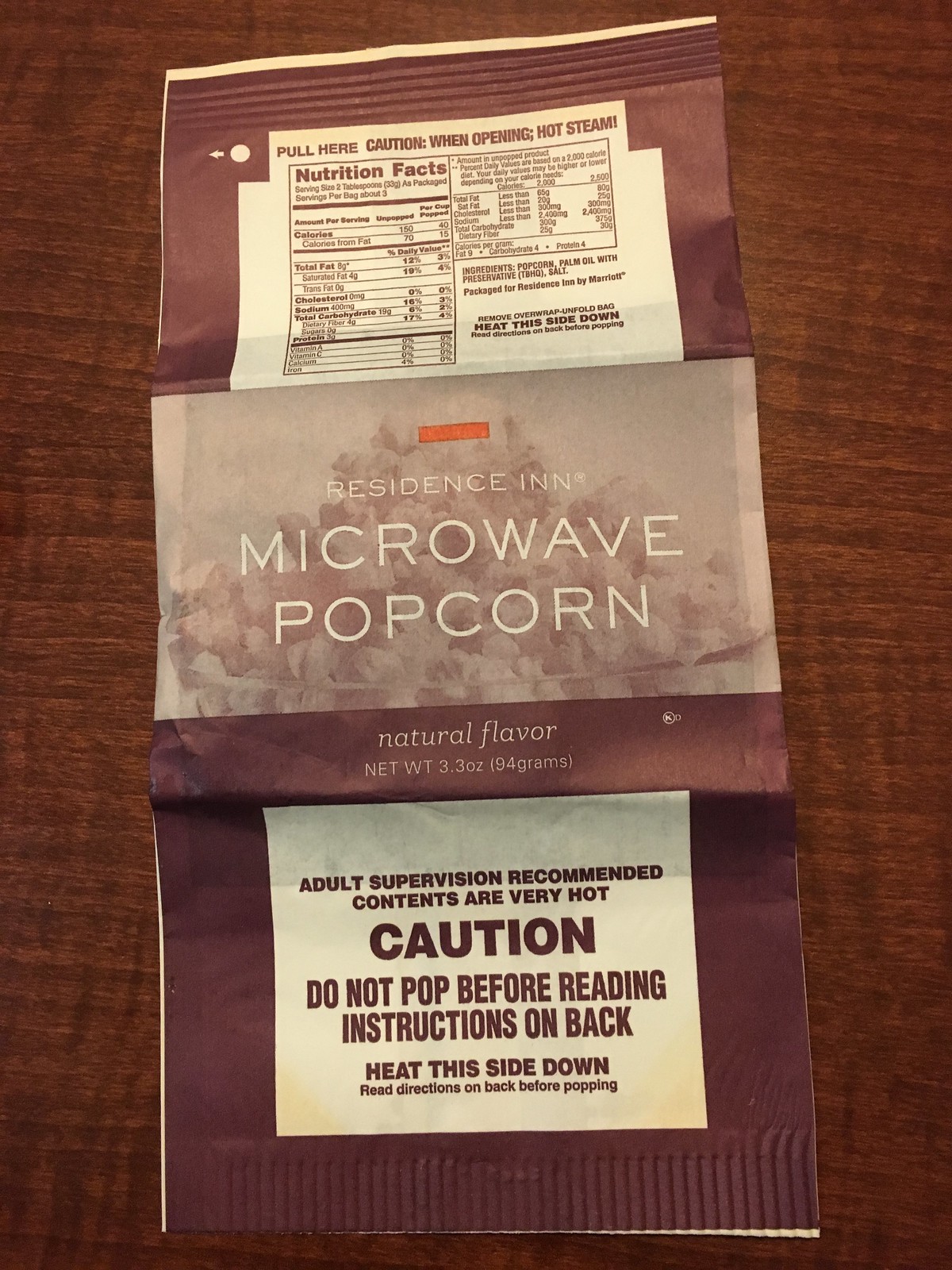On a brown wood laminate countertop, there's an opened package of microwave popcorn. The packaging features an orange rectangle at the top with the brand name "Resident Sin" prominently displayed. Below the brand name, the text reads "Microwave Popcorn" and "Natural Flavor," followed by "Net Weight 3.3 ounces (94 grams)." At the center of the packaging is a large white square containing several cautionary messages: "Adult supervision recommended," "It's very hot," and "Caution: Do not pop before reading instructions on the back." Additional instructions on the white square include "Heat this side down," "Read directions on the back before popping," and "Pull here, caution when opening." The surrounding areas of the packaging are brown, with another white square at the top indicating the location to pull open the package, along with a section listing the nutrition facts.